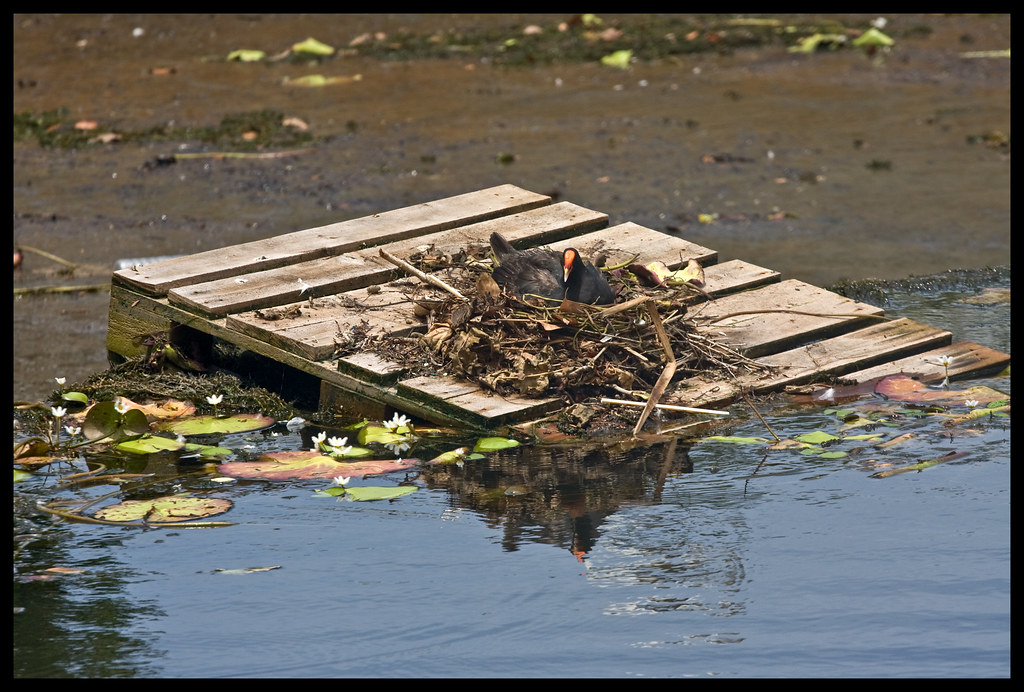In this photograph, we see a close-up of a wooden pallet, possibly a fragment of an aged dock, washed up on the muddy shore of a lake. Surrounding the pallet, the murky water is dotted with blooming lily pads and various pieces of floating trash. On this makeshift raft, a bird, resembling a black duck with an orange head, has constructed a large nest from an assortment of sticks, leaves, twigs, and debris. The bird is perched in its nest, likely incubating eggs. The scene is framed by a partially wet, dark brown beach, scattered with stones, dead leaves, and other natural debris. The overall impression is one of a resourceful bird making the best of a dingy, polluted environment.